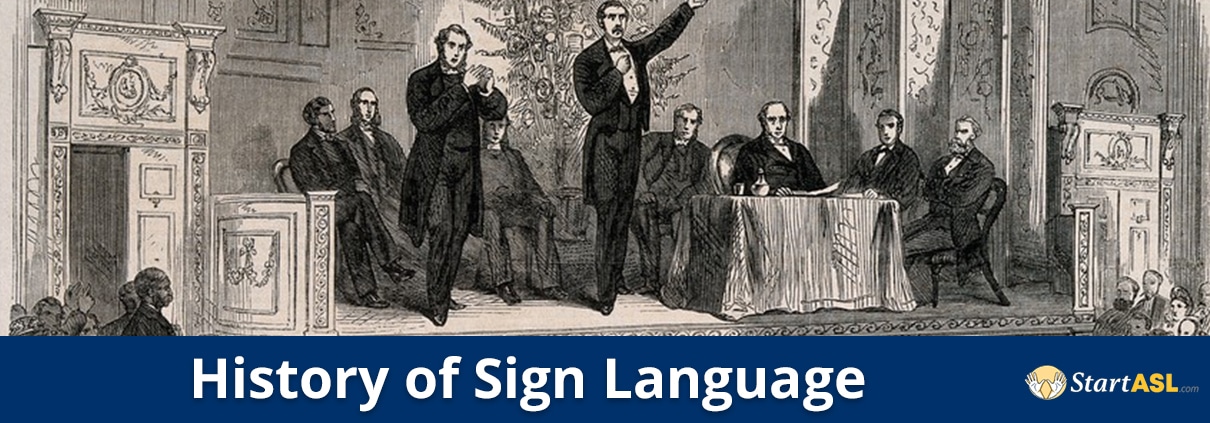The poster is designed as a banner with an intricate, old-fashioned illustration occupying the upper portion. The artwork depicts a historical scene featuring a group of men; two are standing prominently at the front, while approximately seven others are seated. Some of these men are gathered around a small table, and others are positioned to the left. In the background, there is a detailed drawing of a tree, and the wall is adorned with various illustrations. A podium can be seen to the right, suggesting that the scene takes place on a stage. To the left, there appears to be a door and a column with intricate designs.

The lower section of the poster transitions into a blue background with text that reads, "History of Sign Language," alongside "Start ASL." To the right of this text is an emblem featuring two hands within a round yellow circle. The border area of the illustration shows partial views of additional onlookers, emphasizing the focal group's importance. The overall design effectively combines historical imagery with informative text to highlight the subject matter.